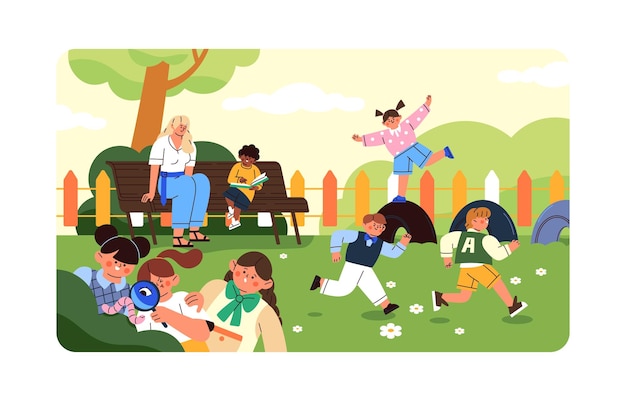In a lively and colorful cartoon park scene, numerous children are thoroughly engaged in various activities. Centrally located, a brown-skinned child is seated on a dark brown bench without armrests, sharing a book with a blonde-haired white woman dressed in a white shirt and blue pants. Behind them, a green bush and a tall tree stand, alongside a distinctive fence made of tipped rectangles in yellow and dark brown hues.

In the bottom left corner, three girls are gathered around a bush, one of them examining a worm with a magnifying glass. Nearby, white flowers dot the vibrant green grass. To the right of the bench, a child joyfully bounces on a partially embedded tire.

The scene also captures two boys energetically running towards the right. Further right, a girl walks across a line of tires embedded in the ground, illustrating the park’s playful nature. The park is vividly rendered with an array of diverse characters in different clothing styles, hair colors, and skin tones, highlighting the rich tapestry of activities and interactions in this charming outdoor setting.